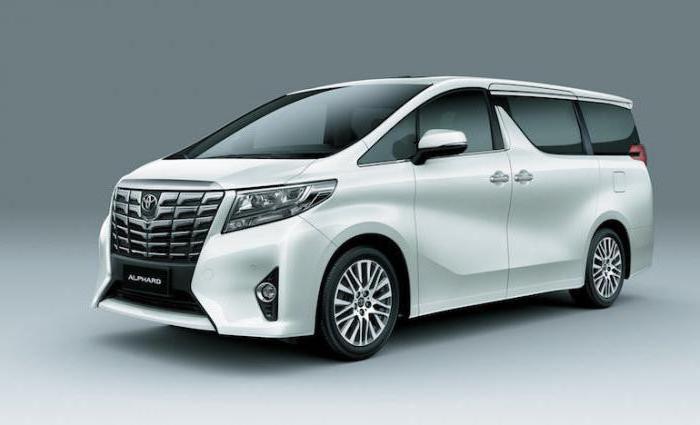This image features a sleek, modern Toyota minivan, likely a 2024 model, with a white or silver exterior. The vehicle has a futuristic, spacey design, featuring clear, rounded headlights and a distinctive grille adorned with multiple square patterns and the iconic Toyota emblem. The van's aerodynamic yet boxy shape is accentuated by its tinted windows and stylized, curved sides. It is equipped with sliding doors and black accents that enhance its contemporary look. The gas tank is located on the left side of the minivan, which is photographed against a gray background, giving it a sharp, promotional appearance akin to stock images used in car advertisements. The minivan exudes a swanky, cutting-edge aesthetic, suitable for showcasing the latest advancements in automotive design.